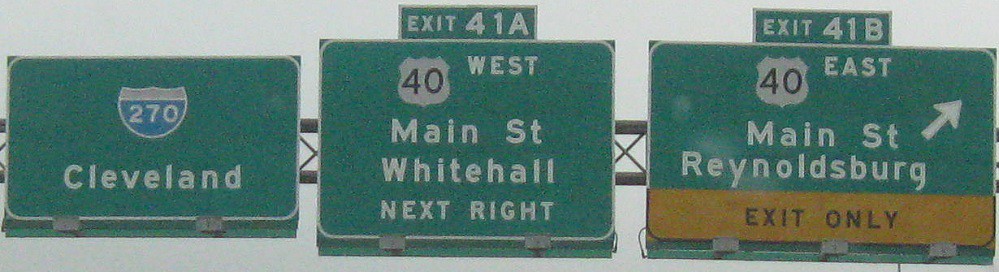The image captures a view from above an interstate featuring three prominent green directional signs against a light gray sky. 

1. The leftmost sign displays the Interstate 270 shield with a blue background, directing travelers towards Cleveland.

2. The middle sign, labeled "Exit 41A," includes an additional rectangular section at the top. It indicates Route 40 West, leading to Main Street and Whitehall, with instructions for the next right turn.

3. The rightmost sign, marked "Exit 41B," also features a similar top section. It guides drivers onto Route 40 East towards Main Street and Reynoldsburg, with a diagonal arrow pointing to the right. Below this, a bright yellow section cautions "Exit Only" in bold black letters.

Each element is clearly detailed, ensuring drivers can navigate easily from the busy interstate.